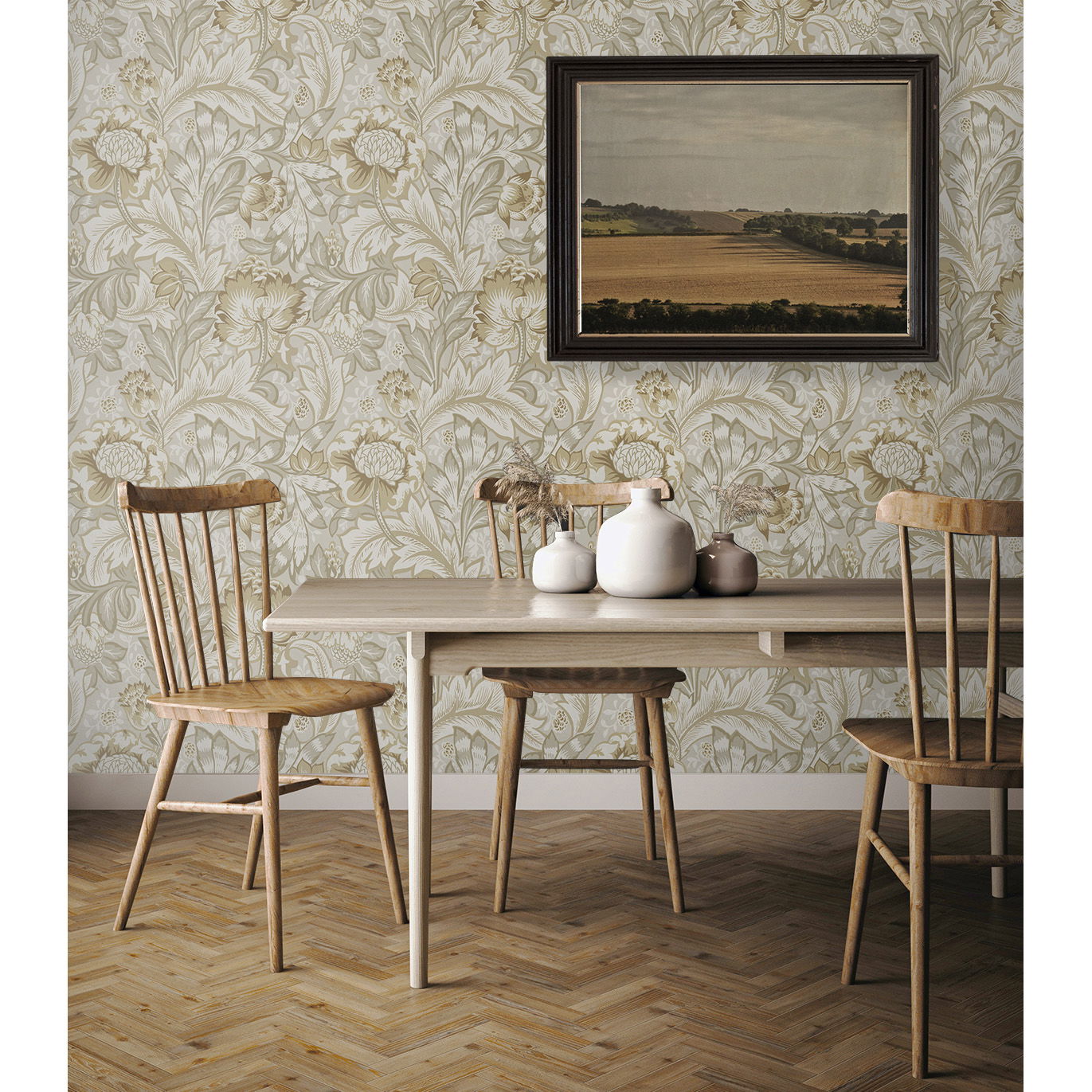The image depicts a cozy dining room with a charming rustic ambiance. At the center is a long, slender dining table made of white ash wood, surrounded by three light-colored wooden chairs arranged with one chair behind, one to the side, and one in front of the table, all facing towards it. The table serves as a display for three vases of varying colors—light grey, white, and brown—serving as an elegant centerpiece. One of the vases is adorned with tall wild grass, adding a touch of nature to the setting. The floor is covered in a geometrical wood pattern, providing a harmonious continuation of the wooden elements throughout the room. The wall is decorated with a flowery patterned wallpaper in light and dark yellows and creamy whites, and prominently features a framed artwork. This painting, enclosed in a black frame, illustrates a serene farm scene with a field of wheat bordered by trees, under a clear sky.